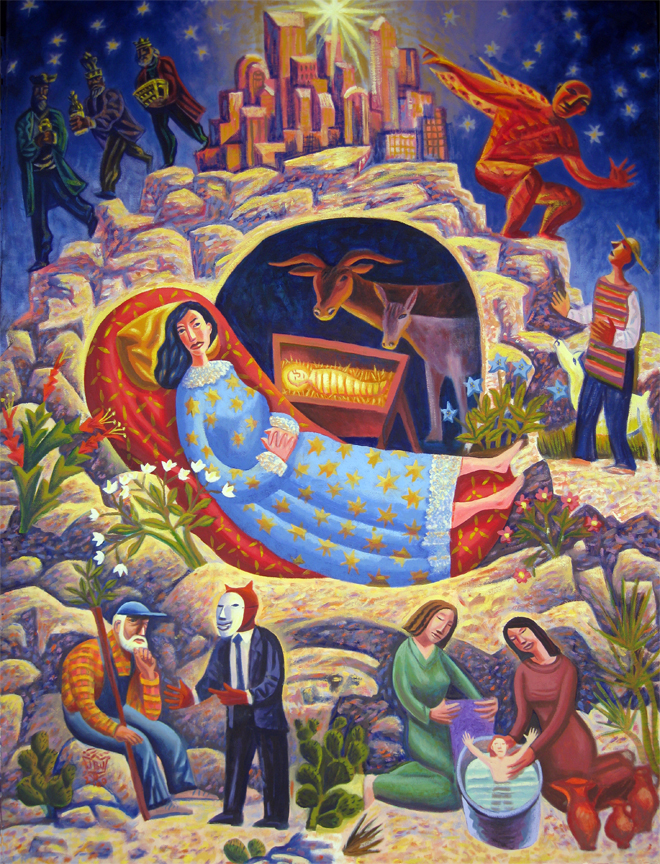This vibrant, surrealistic artwork depicts a vivid nighttime scene brimming with rich, detailed elements. The background showcases a deep blue night sky adorned with yellow stars. Dominating the top of the image is a rocky mountain, on which stands an orange castle emitting a radiant star. Situated on the right side of the mountain is an orange figure that appears to be on fire, leaping downward. On the left side, three men clad in long coats and striped pants—blue and black, yellow and black, and green, respectively—march uphill, carrying a gold treasure chest and a bottle. They sport distinctive crowns.

In the center of the mountain, two mules gaze upon a glowing infant wrapped in swaddling clothes within a brown manger, suggestive of baby Jesus with a halo-like bright light above his head. Below the mules, a woman in a blue dress adorned with yellow stars reclines on a long orange and yellow chair. Her dark hair cascades around her amidst scattered rocks and stones.

The lower section of the image features various interactions: on the left, a farmer sits on a rock, conversing with a devilish figure in a white mask and suit, who holds a large stick or plant. On the right, two women bathe an infant in a silver pot. The entire composition includes contrasting elements such as disjointed cityscapes, stylized skyscrapers, and tunnel-like structures within the mountain, blending reality with imaginative juxtapositions. The color palette is a striking mix of blues, yellows, oranges, greens, blacks, and grays, contributing to the overall surreal atmosphere of the scene.